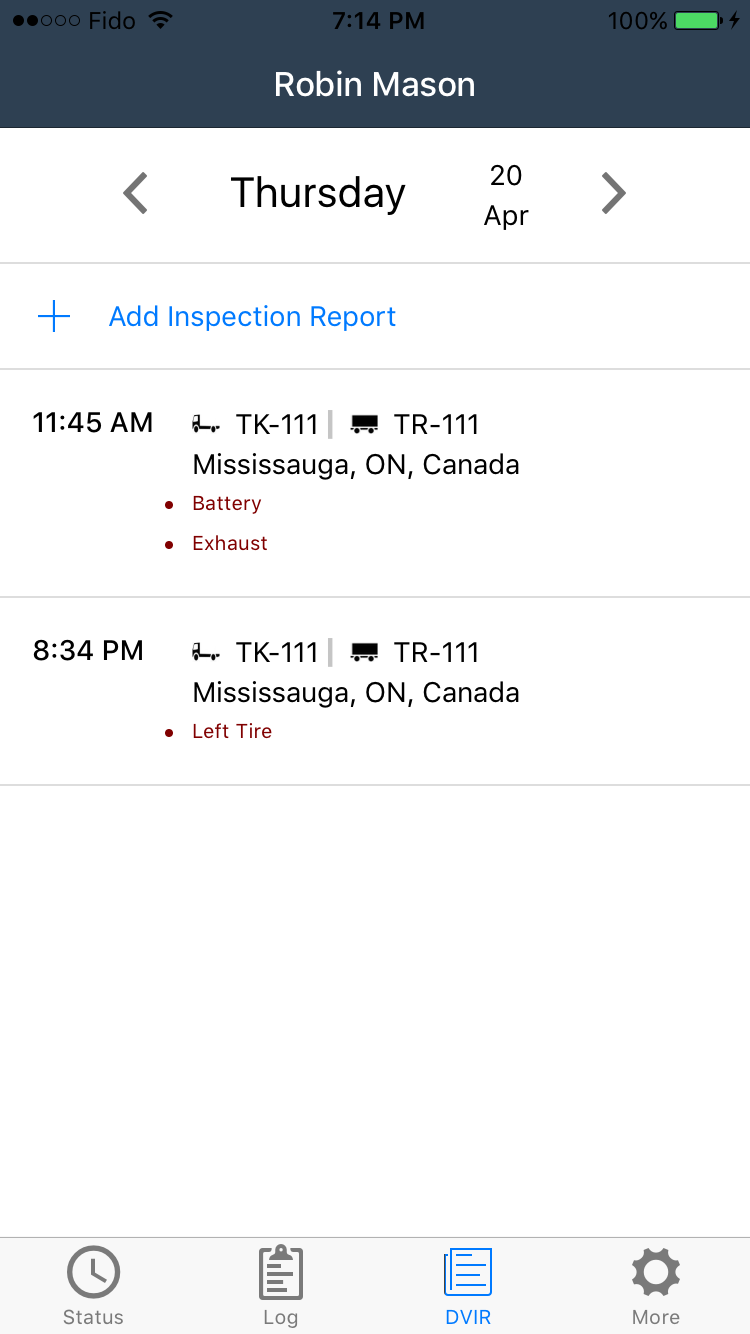This screenshot, likely taken from a mobile phone, provides an overview of various status indicators and contains detailed information related to a vehicle inspection report. 

At the top, a dark purple bar displays the carrier name "Fido," alongside a full Wi-Fi icon and signal bars. The time "7:14 PM" is prominently shown in the center, while the upper right corner indicates a full battery with 100% charge.

Beneath this top section, the text "Robin Mason" is displayed in white font. The interface then transitions to what appears to be a document or form interface. The document header shows the date "Thursday, 20 April" in white on a dark background.

Next, a blue-font command "Plus Add Inspection Report" stands out against the white page, providing the user with an actionable link. Below, in black font, the time "11:45 AM" is recorded, followed by a truck icon labeled "TK-111" and a trailer icon labeled "TR-111." The location "Mississauga, Ontario, Canada" is also noted, followed by a mention of "Battery and Exhaust."

A subsequent entry shows another time stamp "8:34 PM," with the same truck (TK-111) and trailer (TR-111) icons, and the same location. This entry mentions "Left Tire," indicating another point of inspection or issue logged.

The screenshot thus captures essential details of a mobile-based vehicle inspection log, featuring timestamps, vehicle identifiers, and specific inspection items.